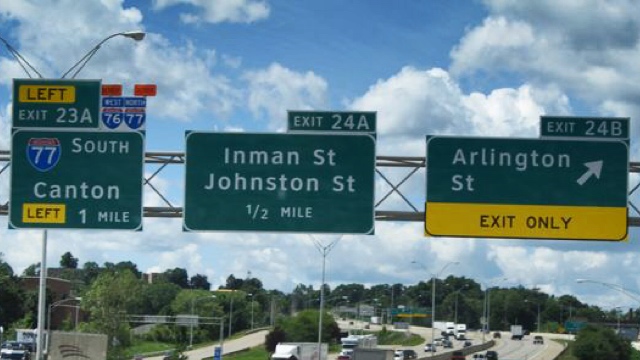This detailed color photograph captures a U.S. interstate highway scene, with a trio of exit signs prominently displayed above the freeway. These signs are mounted on a sturdy metal structure. On the left, the sign indicates "I-477 South to Canton." The center sign directs to "Inman Street, Johnson Street," mentioning it is half a mile ahead and marked as Exit 24A. The rightmost sign informs drivers about "Arlington Street," labeled as Exit 24B, and emphasizes that this lane is for exit only. Below these signs, the interstate is bustling with a diverse array of vehicles. The sky above is brilliantly blue, adorned with fluffy cumulus clouds. Surrounding the highway are patches of lush green trees, extending along the sides and into the distance, enhancing the scenic route.